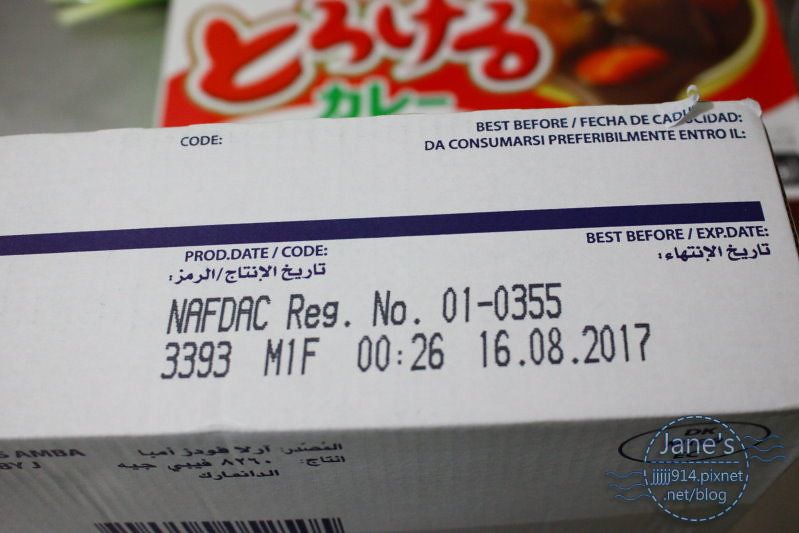This image shows a white package prominently featuring a blue stripe down the middle, which reads "best before" followed by an expiration date. At the top left, the phrase "Code, best before" is present along with its translations into other languages. Below this, there is a hand-written note and a barcode. The text "NAFDAC reg number 01-0355" is printed in large, clear letters. Beneath this are the numbers "3393 M1F00:26/1608/2017." The bottom right corner features a logo within a circle, stating "Jane's Pixnet.net/blog." The background is blurred but reveals a red and white package with some indiscernible Asian writing and what appears to be a brownie.